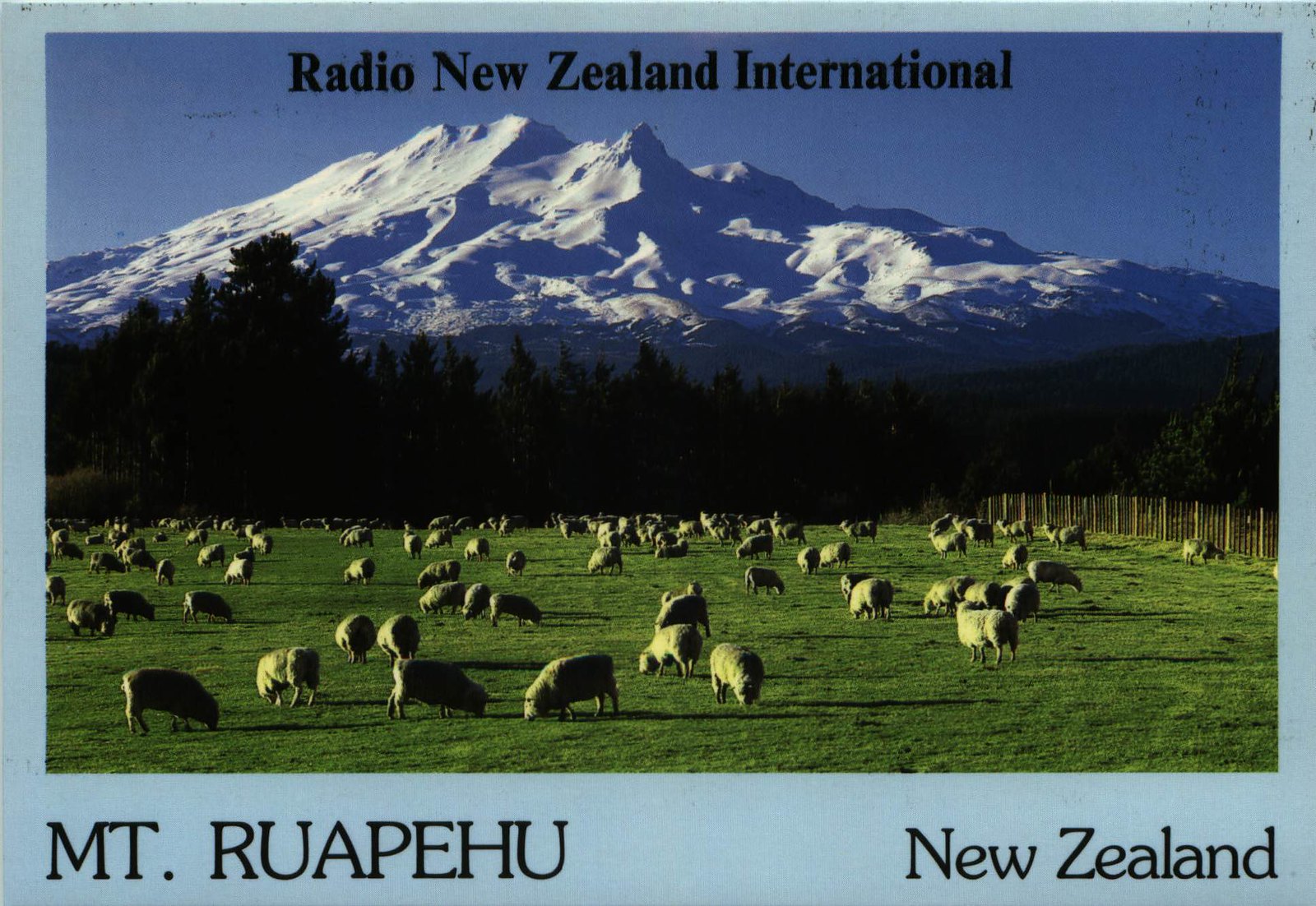This vibrant postcard advertisement for New Zealand features a picturesque landscape, dominated by the majestic, snow-capped Mount Ruapehu towering in the background. In the mid-foreground, there's a dense forest of trees, creating a lush green barrier at the base of the mountain. The foreground is an expansive, verdant pasture dotted with numerous sheep grazing on the green grass, some close to the viewer and others scattered throughout the field, with a fenced area enclosing them on the right side. The postcard has a blue border, with the text "Mount Ruapehu" on the bottom left and “New Zealand” on the bottom right. Prominently displayed at the top center in black letters is the phrase "Radio New Zealand International," inviting viewers to explore the idyllic scenery. The main colors of the image are blue, green, black, and white, emphasizing the natural beauty of the landscape.